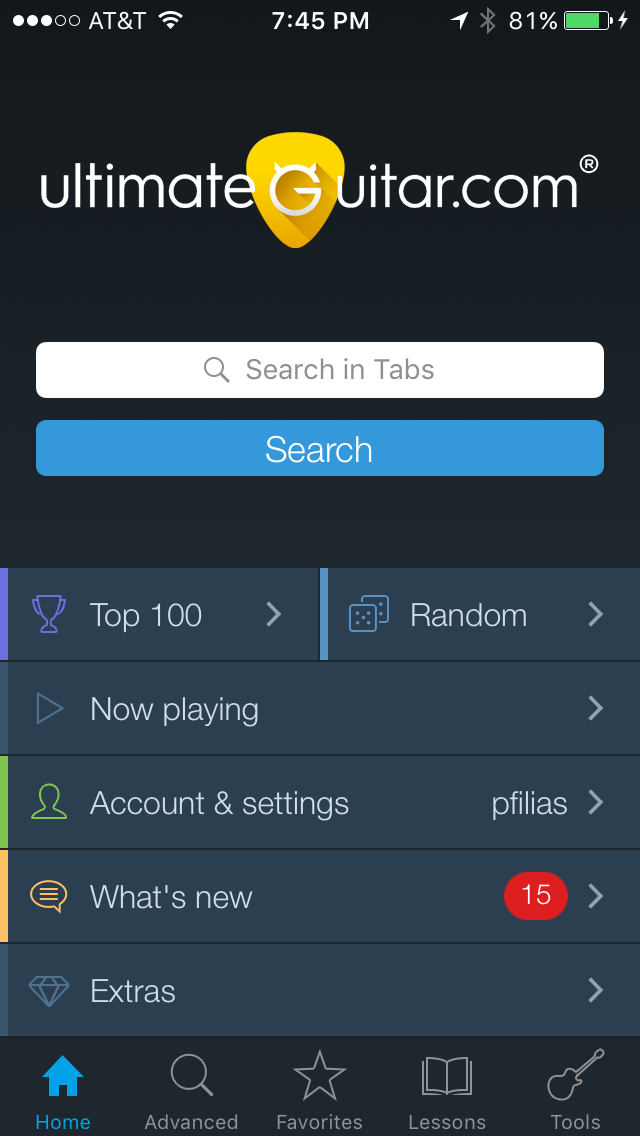The image is a detailed screen capture from a cell phone displaying the UltimateGuitar.com app interface. At the very top of the screen, the status bar shows typical icons such as the AT&T signal, the current time, and a battery indicator with a green segment illustrating the charge level. Below this, against a black background, the app's logo is prominently featured: “ultimate guitar dot com” in white lettering, with a yellow guitar pick positioned behind a large white 'G'.

The central part of the screen features a white search bar with grey tabs followed by a blue search button. Directly beneath the search bar is a menu on a grey background that includes several options: "Top 100," "Random," "Now Playing," "Account and Settings." Positioned under this menu is a section labeled "What's New," which has a notification indicator showing the number 15. Following that is another section labeled "Extras."

At the very bottom of the screen, there is a black navigation bar with typical cell phone navigation buttons: home, advanced, favorites, lessons, and tools. The layout is centrally aligned, with the yellow guitar pick logo being a focal point in the top center, and the rest of the menu options cascading down from there. The color palette of the interface incorporates a range of hues, including lighter and darker blues, yellows, green, red, and white, creating a vibrant and easily navigable display.